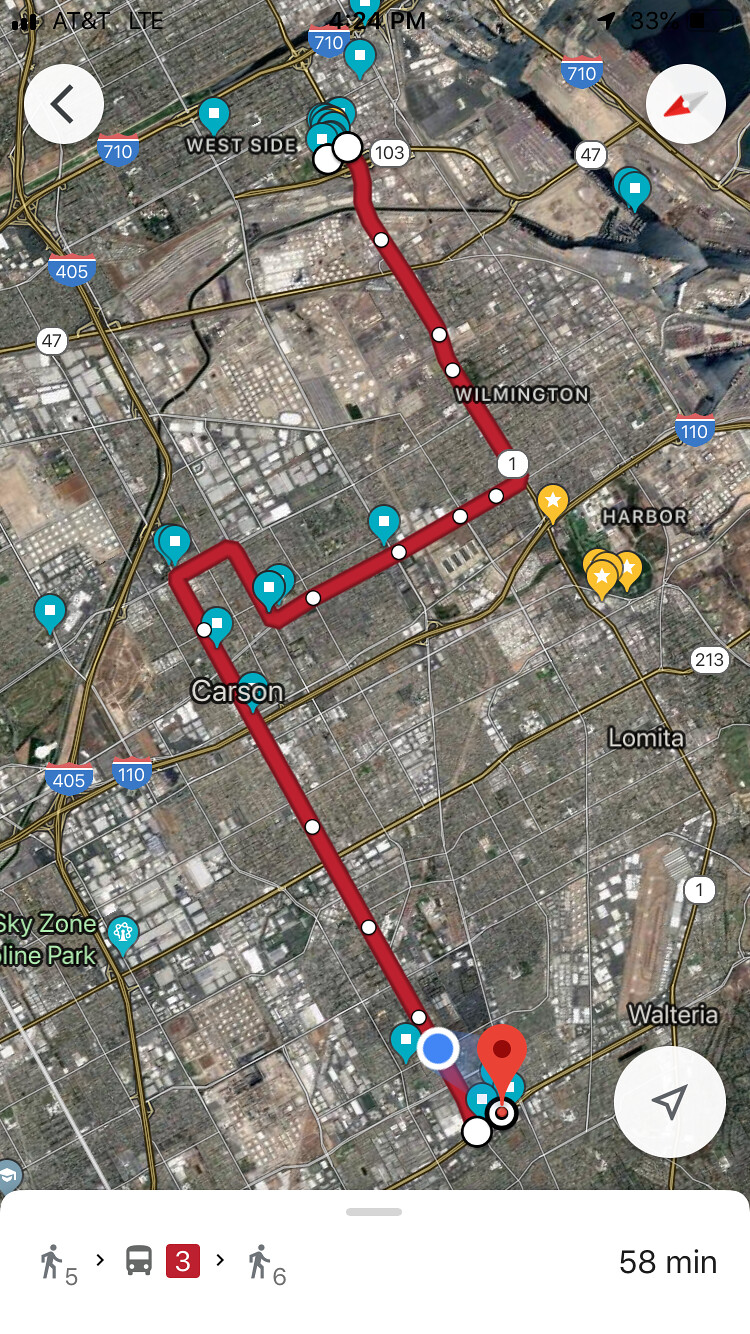The image depicts a smartphone screen displaying a detailed map. A compass icon is visible, indicating the orientation and directions of the map. The plotted route begins in the lower right-hand corner, zigzagging diagonally upwards to the right, dipping slightly downward, then proceeding horizontally to the right, and finally moving upwards until it reaches the destination. The journey is estimated to take 58 minutes. 

The map features several city names including Wilmington, Westside, Carson, Lomita, and Harbor. Major roads and highways shown include Route 103, Route 1, Interstate 405, and the continuation of Interstate 405 into Interstate 710. Various markers representing businesses and other points of interest dot the route. A prominent "back" button is also displayed, allowing users to return to the previous screen.